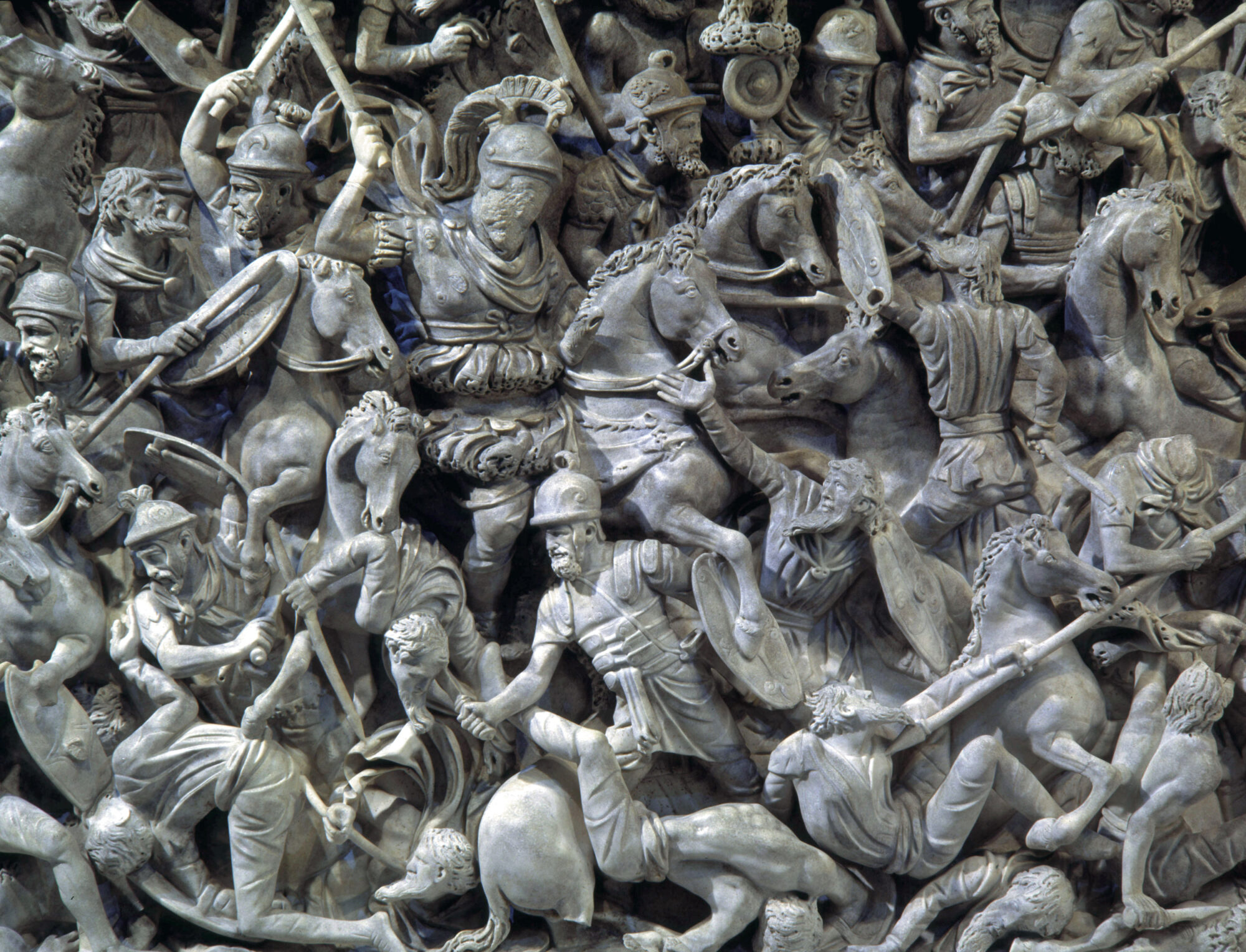The image depicts a detailed marble sculpture capturing a chaotic ancient or early medieval battle scene. Positioned centrally, it features a dramatic array of Roman or similar soldiers and horses intricately carved in shades of white and grey, with subtle reflections suggesting an outdoor display. In the heart of the composition, a helmeted man atop a horse swings an axe or similar weapon, though the top of the weapon is cut off. Surrounding him are other mounted and foot soldiers, all clad in armor, wielding swords, pikes, shields, and scythes. These figures are densely packed, intensifying the scene's chaotic nature. Despite the lack of text, the sculpture's depth is palpable, almost three-dimensional, underlined by the contrasting hues and light play, with faint bluish tones accentuating the predominantly grey palette.